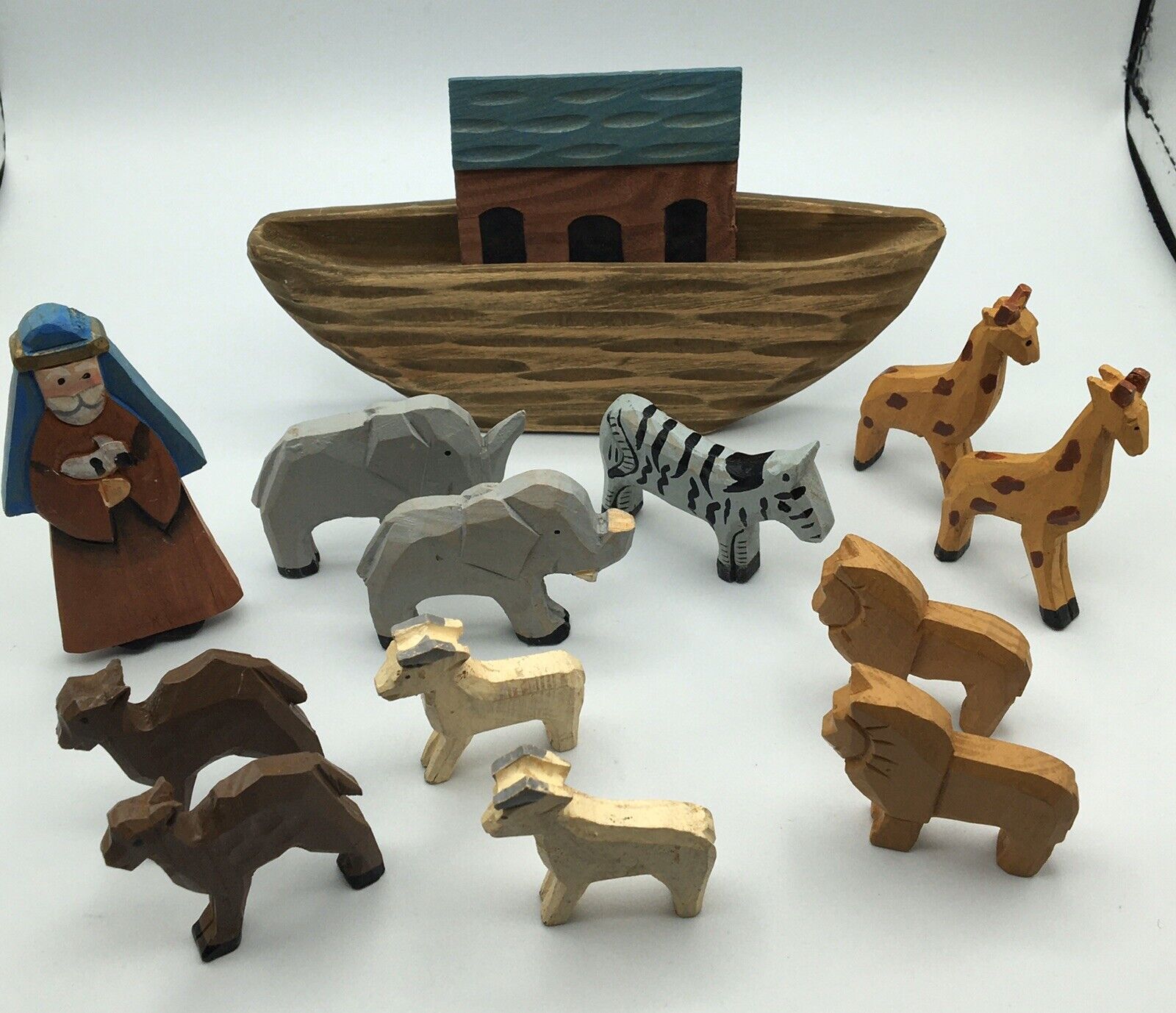The rectangular image, slightly wider than it is tall, showcases an intricately detailed, wooden carved set depicting the scene of Noah's Ark against a neutral beige-gray background. At the center, Noah stands wearing a brown robe and a blue head covering, gently holding a lamb. The Ark itself, crafted from dark wood with lighter streaks and resembling a ship, sits prominently in the back with a cabin featuring three arched doorways and a green roof. The array of painted wooden figures includes pairs of elephants, giraffes, lions, camels (or potentially horses), and goats, all meticulously placed around Noah. A solitary zebra stands out among the pairs. The entire scene is a harmonious assembly of delicate craftsmanship, vibrant colors, and thoughtful arrangement, bringing the biblical tale to life.